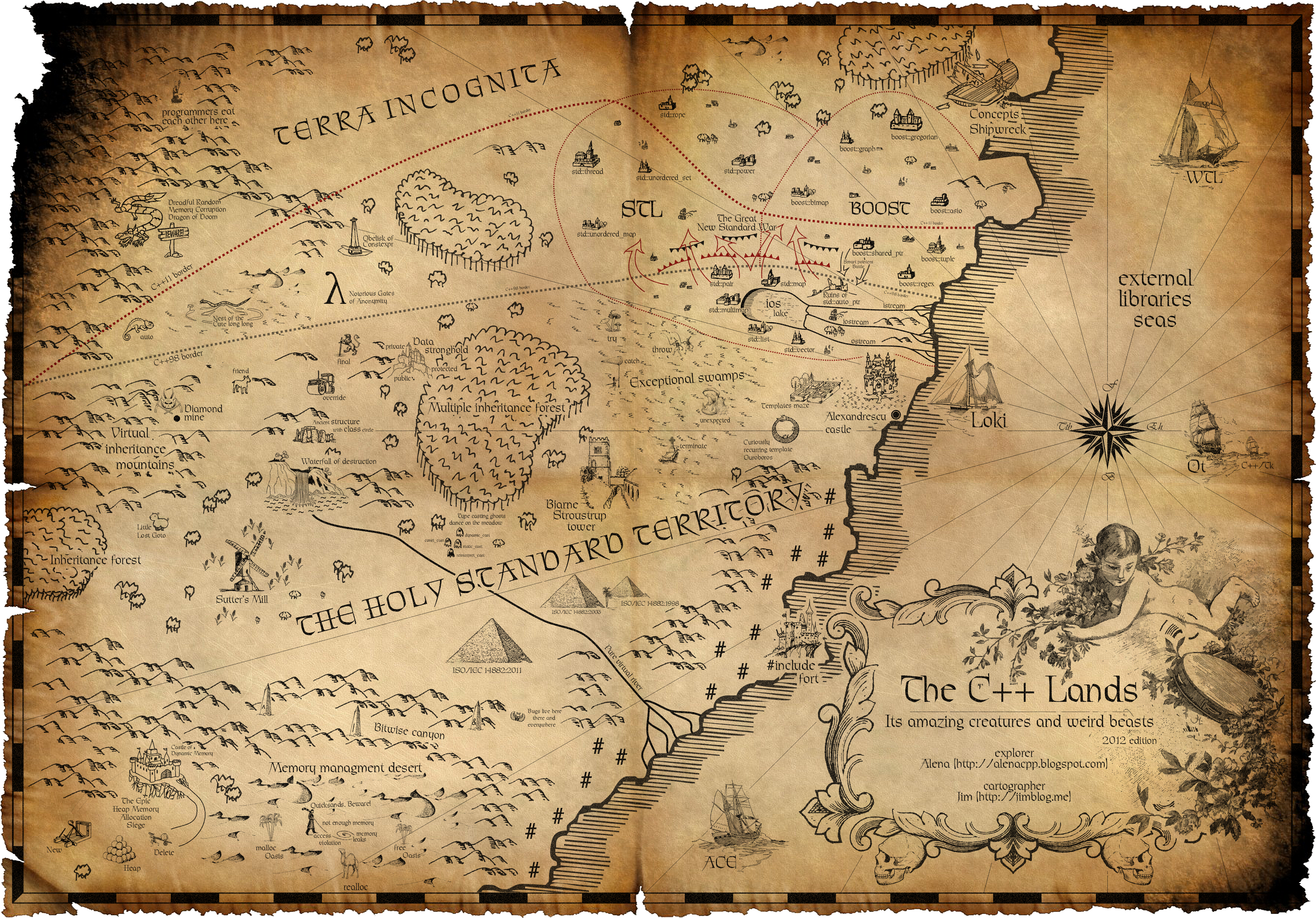This detailed caption could comprehensively describe the image:

---

A meticulously folded paper map is the focus of this image. The map, although designed to appear antique with its light tan color and artfully burnt edges, is actually of modern creation. The scorched borders, which transition into a charred black, give it an aged and rugged appearance, complemented by jagged, torn sides.

Prominently displayed across the map in bold lettering are the words "The Holy Standard Territory" and "Terra Incognita," denoting unexplored or unknown lands. The oceanic sections of the map are illustrated with vintage ships sailing upon the waters, adding to the historical aesthetic.

In the bottom section, a legend reads "The C++ Lands," hinting at a whimsical or fantastical interpretation of programming territories. The legend also mentions "Amazing Creatures and Weird Beasts," attributed to an explorer named Alina, directing viewers to a blog at 'http://alenaCpp.blogspot.com' for more information. 

Calligrapher Jim is credited for the map's artistic details, with an additional reference to his work at 'http://filmblog.me,' dated 2012. Within the waters, enigmatic labels such as "External Library," "Oat," or "Qt," "LLK E Looky," and "Acy," are scattered, adding an element of mystery and inviting further exploration.

---

This caption provides a thorough visual description, enhancing the viewer's understanding and imagination about the map.